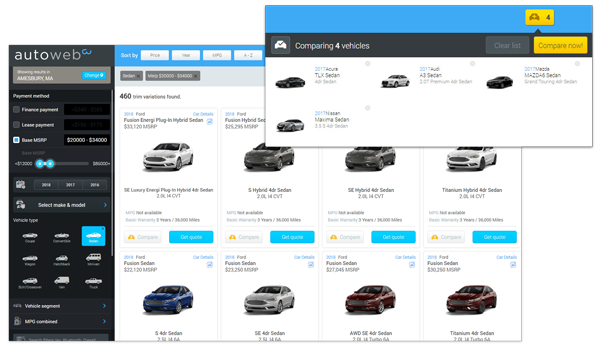This detailed screenshot from AutoWeb.com showcases its car comparison feature. The focal point is a nested screenshot displaying the comparison of four vehicles, framed by a light blue header indicating the number of cars being compared. Below, a dark gray banner clearly states "Comparing 4 Vehicles" and features two buttons: "Clear List" and "Compare Now." Within this section, four cars are shown, distinguished by their colors: two black, one white, and one silver, though their specific models are not visible.

The larger background screenshot provides a broader view of the website’s layout. On the left-hand side, users can find filtering options against a black background. The top banner displays the AutoWeb logo, followed by a search bar where users can input criteria such as best gas mileage, lease payment, finance options, and vehicle type.

To the right of the filters, the main content area lists 460 cars based on the applied filters. These vehicles, all sedans, come in various colors and are priced between $20,000 to $33,000, averaging around $25,000. Each listing includes a neon blue button for getting a quote. The text on the site uses a color scheme of black, light gray, and light blue, contributing to the clean, user-friendly interface that assists users in comparing different car models effectively.